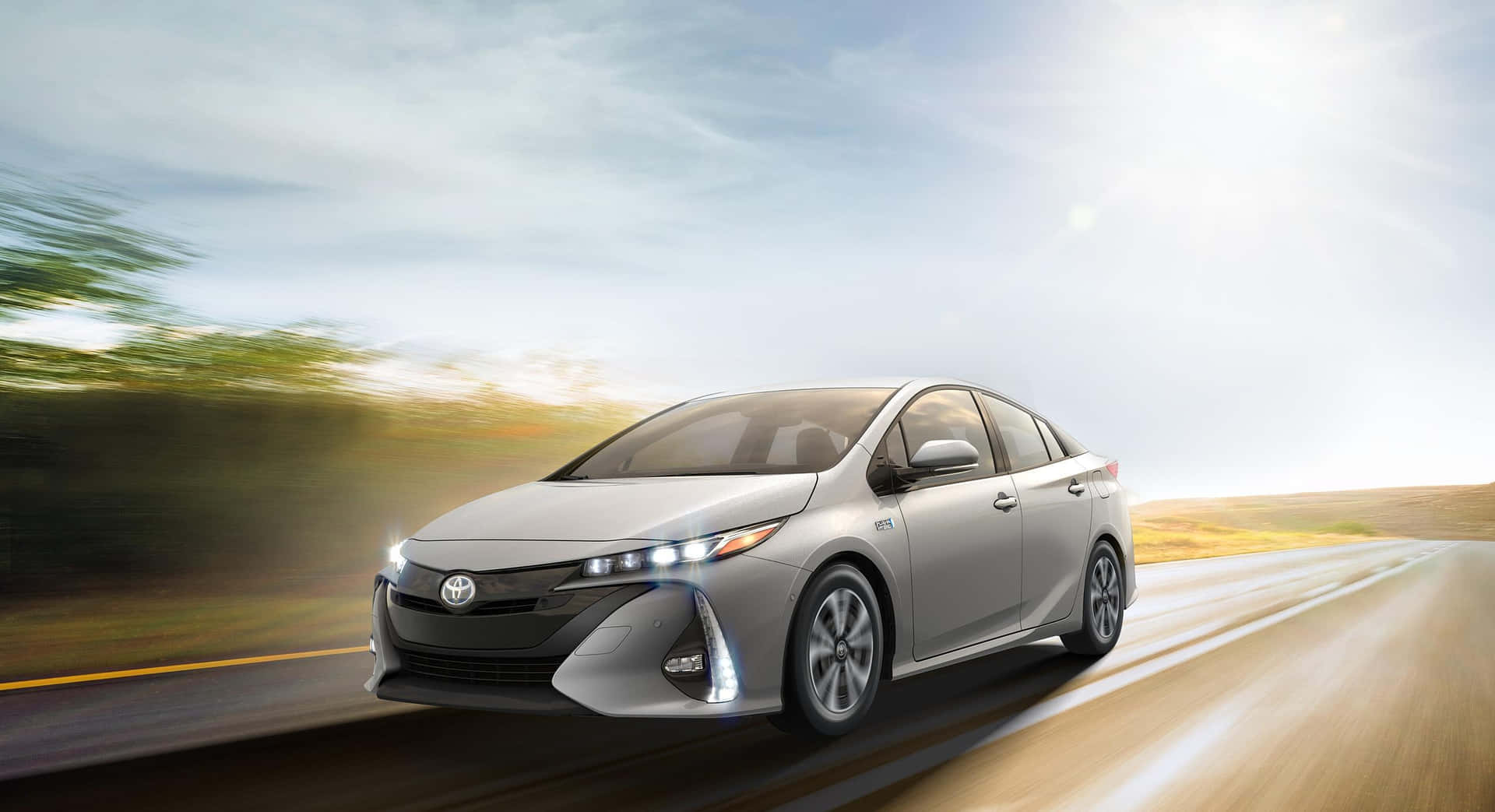This image is a highly detailed rendering of a silver Toyota Corolla, potentially drawn for a car advertisement or brochure. The car, featuring the distinctive Toyota emblem on its front and a black grille beneath it, is depicted in motion, driving towards the bottom left corner of the image. The headlights are on, adding a touch of realism, even though it is a bright day with the sun shining in a light blue sky filled with white clouds.

The car occupies a central position, with its front angled slightly towards the viewer, allowing a clear view of the hood, windshield, driver's side, and part of the passenger side. The passenger side headlight is partially cut off. The road beneath is a typical grey highway, marked with white lines that widen towards the bottom left and narrow into the distance towards the top right.

The background showcases a blend of rural scenery. On the left side of the image, behind the car, are blurred trees or bushes in various shades of green and yellow, suggesting high speed. To the right side of the car, the landscape transitions to open fields of brown and yellow grass, resembling a late autumn countryside. The environment is devoid of buildings and people, emphasizing the car's solitary journey along the rural road.